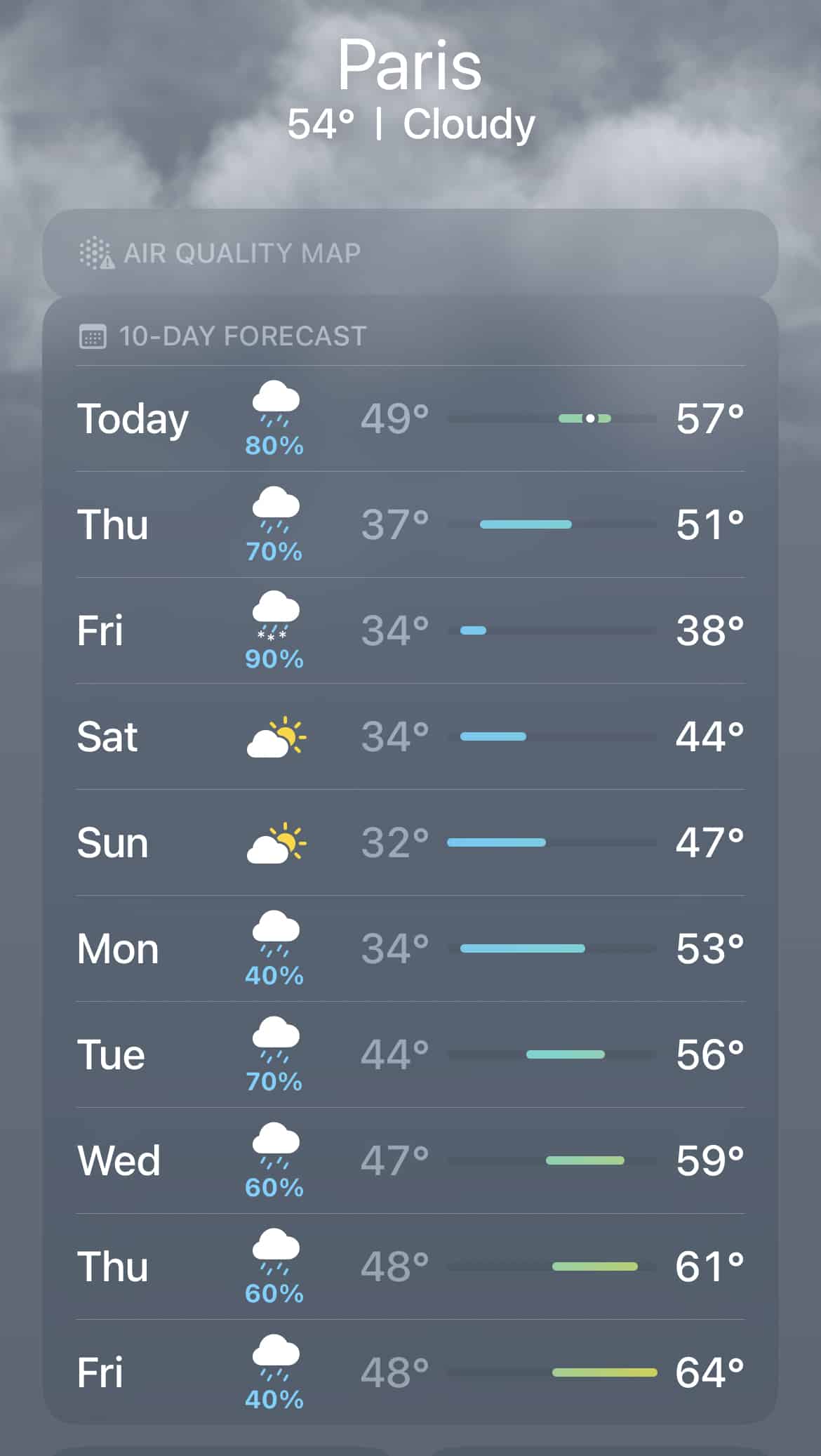In this vertical rectangular image, we are presented with a screenshot that captures a weather forecasting page. The upper third of the background showcases a very cloudy, gray sky, lending a somber tone to the image. The lower two-thirds of the image remain a solid dark gray.

The weather forecast is prominently displayed in the center of the image, spanning ten days, each day listed in a column format. A small calendar icon is situated to the left of the "Ten Day Forecast" heading. The detailed forecast starts with today’s weather, which includes an 80% chance of clouds and rain, with temperatures ranging between 49 degrees and 57 degrees Fahrenheit.

Following that, the forecast for the next days is: 
- Thursday shows a 70% chance of rain.
- Friday has a 90% chance of rain.
- Saturday is predicted to be partly cloudy with periods of sunshine.
- Sunday continues to be partly cloudy with more sun.
- Monday has a 40% chance of rain.
- Tuesday forecasts a 70% chance of rain.

This detailed forecast allows one to anticipate the weather conditions for the upcoming week with considerable clarity.